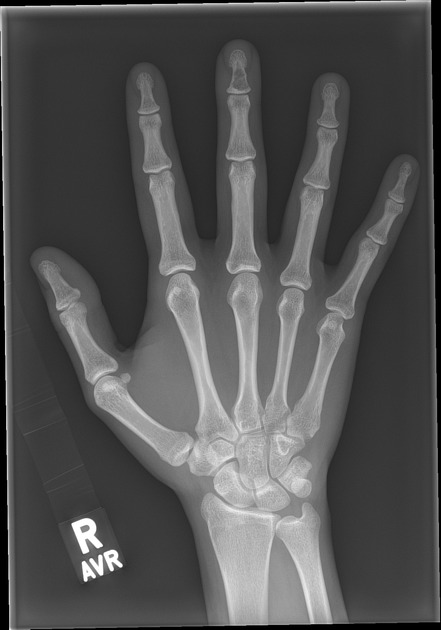This image features a black-and-white x-ray photograph of a human right hand, positioned in a portrait layout with the top and bottom edges shorter than the sides. The hand appears large and occupies the center of the image, which is set against a completely black background. The bones of the hand are stark white, distinctly outlining each of the four fingers and the thumb, all of which are perfectly outstretched and not touching each other. Surrounding the bones is a lighter gray area that indicates the skin. The image is slightly tilted to the left and cuts off just below the wrist. In the lower left-hand corner, white text is visible: a large, bold capital letter "R," and directly beneath it, the initials "A-V-R" in smaller but still bold capital letters. This x-ray shows no signs of damage or additional markings, and there are no rings or other adornments on the hand.